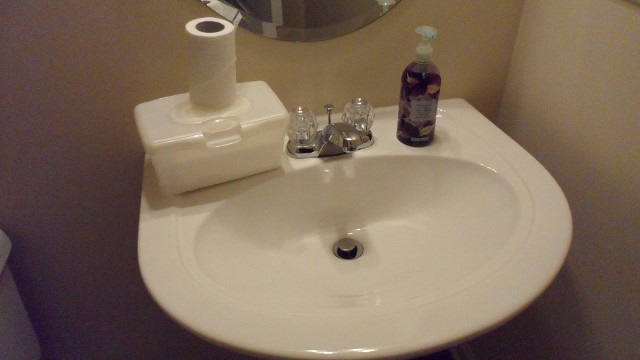The image displays a close-up view of a white porcelain wash hand basin situated in the corner of a bathroom. The basin features a chrome-colored faucet with transparent glass handles for temperature control. On the left side of the faucet rests a white plastic container, likely holding sanitary wipes, with a partially used roll of white toilet paper placed on top. To the right of the faucet stands a clear plastic pump bottle filled with purple liquid, presumed to be hand wash soap. Above the faucet, the lower part of a round-framed mirror is visible, completing the scene.